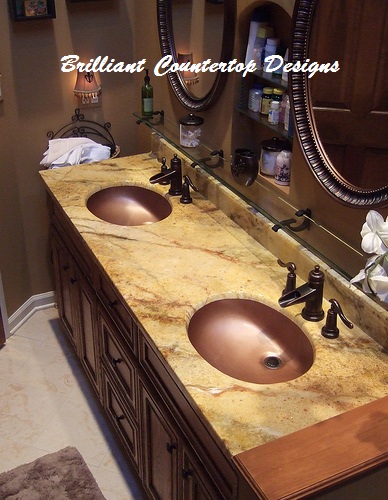The image showcases an elegantly designed bathroom countertop that highlights modern aesthetic sensibilities. The text within the picture reads "Brilliant Countertop Design." The countertop itself is a yellow marble-like Corian material, extending over cabinetry made of natural wood in a warm, wood-tone finish. 

Central to the countertop are two copper-colored sinks, each architecturally sunk into the surface. Complementing the sinks are contemporary, dark copper spigots, featuring individual hot and cold water controls on either side of the straight-out water spout.

Mounted on the wall above each sink are two oval, framed mirrors positioned in alignment with each sink. Between these mirrors, there's an indented section of the wall serving as a medicine cabinet for additional storage. Above the countertop and just in front of the mirrors, glass shelves are installed. These shelves hold various items including a container filled with Q-tips, another storage container, and a bottle of soap with a push spout dispenser.

The bathroom floor is covered with vinyl tiles, providing both durability and easy maintenance. The walls are painted a rich, dark tan color, adding a grounding contrast to the lighter countertop. Additional detail in the room includes a small wall-mounted lamp, whose soft light enhances the overall ambient atmosphere. Absent from view are any electrical outlets. Visible on the right edge of the picture is a vase of white flowers, adding a touch of natural elegance to the space.